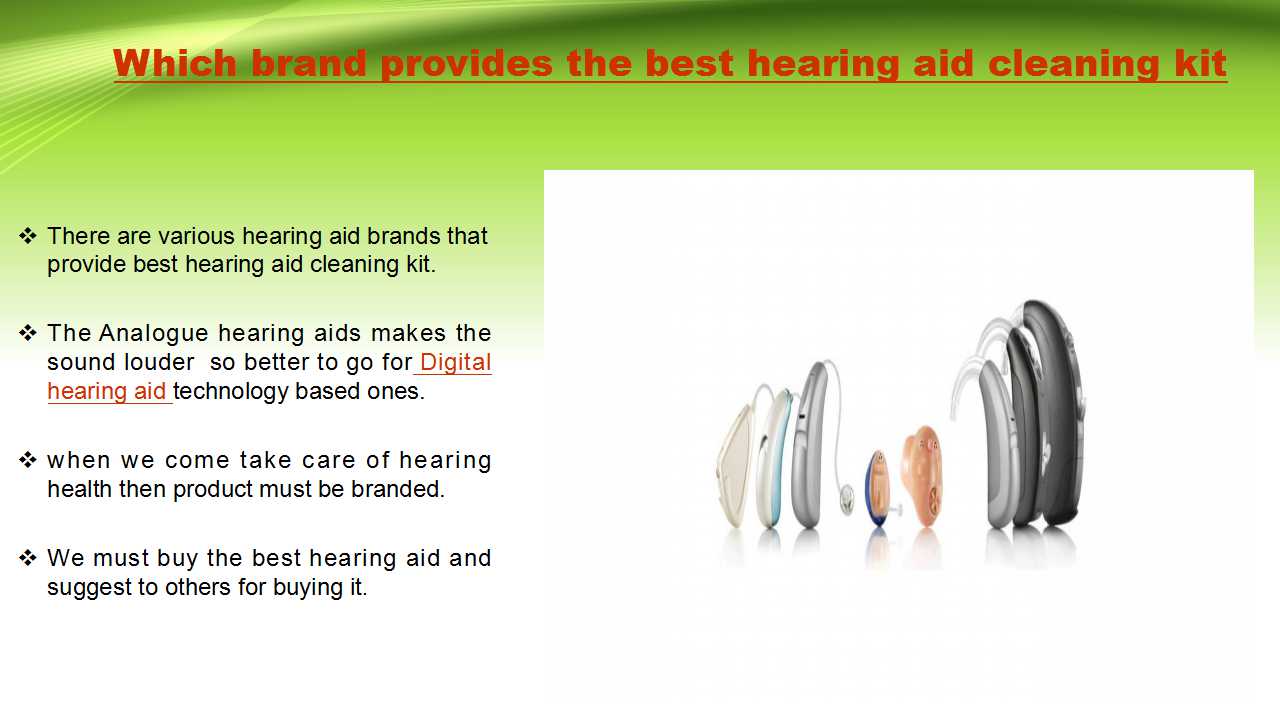This is a detailed advertisement diagram with a gradient background that transitions from pale green at the top to white at the bottom. Prominently displayed in large red text at the top, it reads, "Which brand provides the best hearing aid cleaning kit?" Below the text, set against a white background, is a photograph showcasing a collection of different hearing aids. The hearing aids are presented standing upright in profile: three gray, two white, and two skin-colored or light pink. To the left of the photograph, there are four bullet points in black text that state: 

1. "There are various hearing aid brands that provide the best hearing aid cleaning kits."
2. "Analog hearing aids make the sound louder, so it is better to go for digital hearing aid technology-based ones."
3. "When we take care of hearing health, the product must be branded."
4. "We must buy the best hearing aid and suggest it to others for purchase."

Overall, this diagram serves as an informative advertisement emphasizing the importance of using branded, high-quality hearing aids and cleaning kits, and it suggests opting for digital over analog technology.